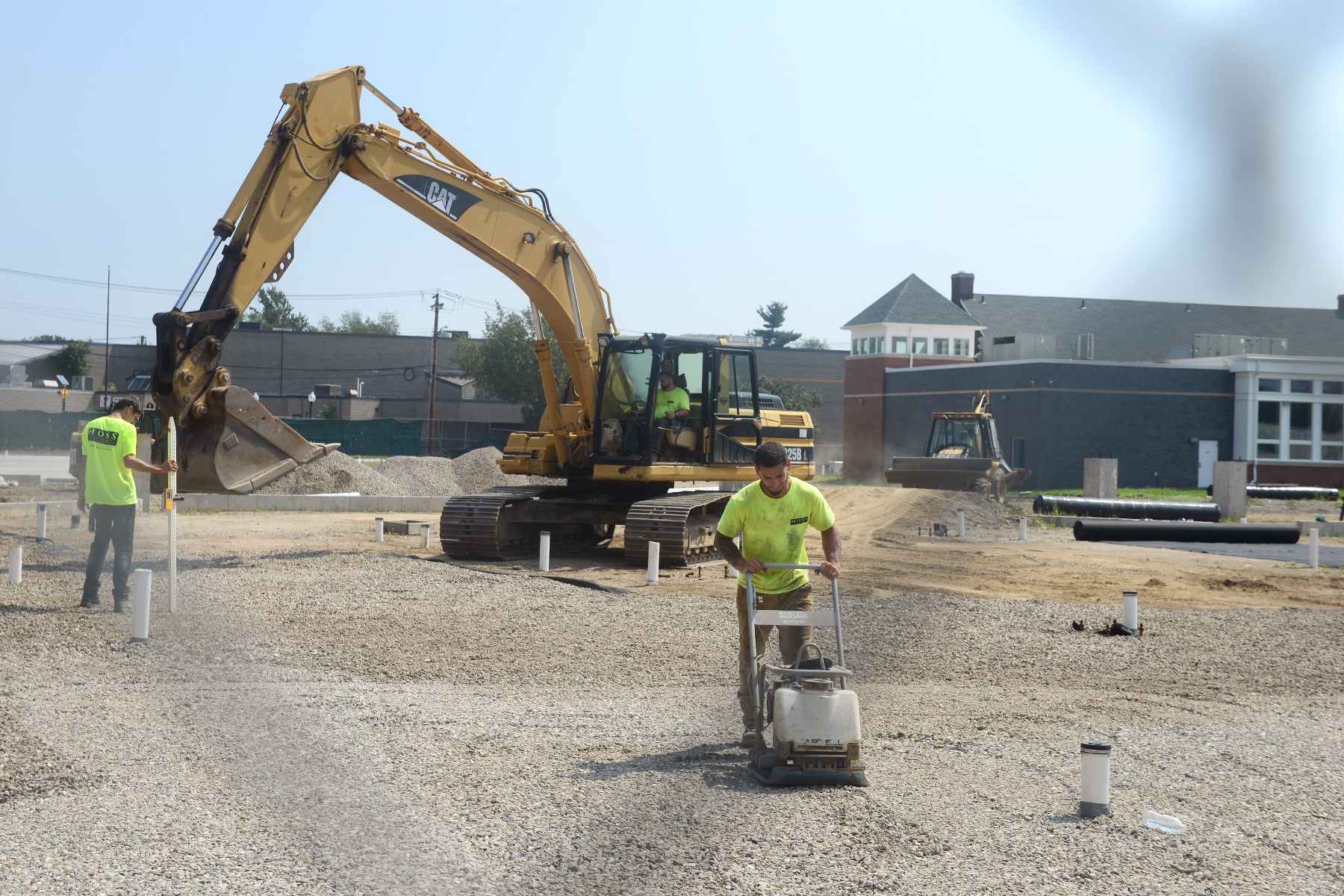The photograph captures a bustling construction site featuring three individuals, all clad in neon yellow shirts and pants for high visibility. At the center, a worker is operating a machinery, possibly designed to flatten the ground or remove small rocks. Just behind him, another worker is stationed inside a large CAT backhoe, diligently operating the machine to excavate or move dirt. To the left, the third worker is standing near the neck of a crane, meticulously placing markers, perhaps for measurement purposes or guiding the machinery operation. The scene unfolds on a gravel lot, with numerous pipes scattered around, suggesting future groundwork for utilities. In the background, a partially visible building with a castle-like top is set against the sky, hinting at the construction's commercial nature—potentially the development of new stores, as evidenced by the surrounding structures. The entire scene is slightly blurred by a chain link fence, adding a gritty, realistic filter to the depiction of hard labor and development.